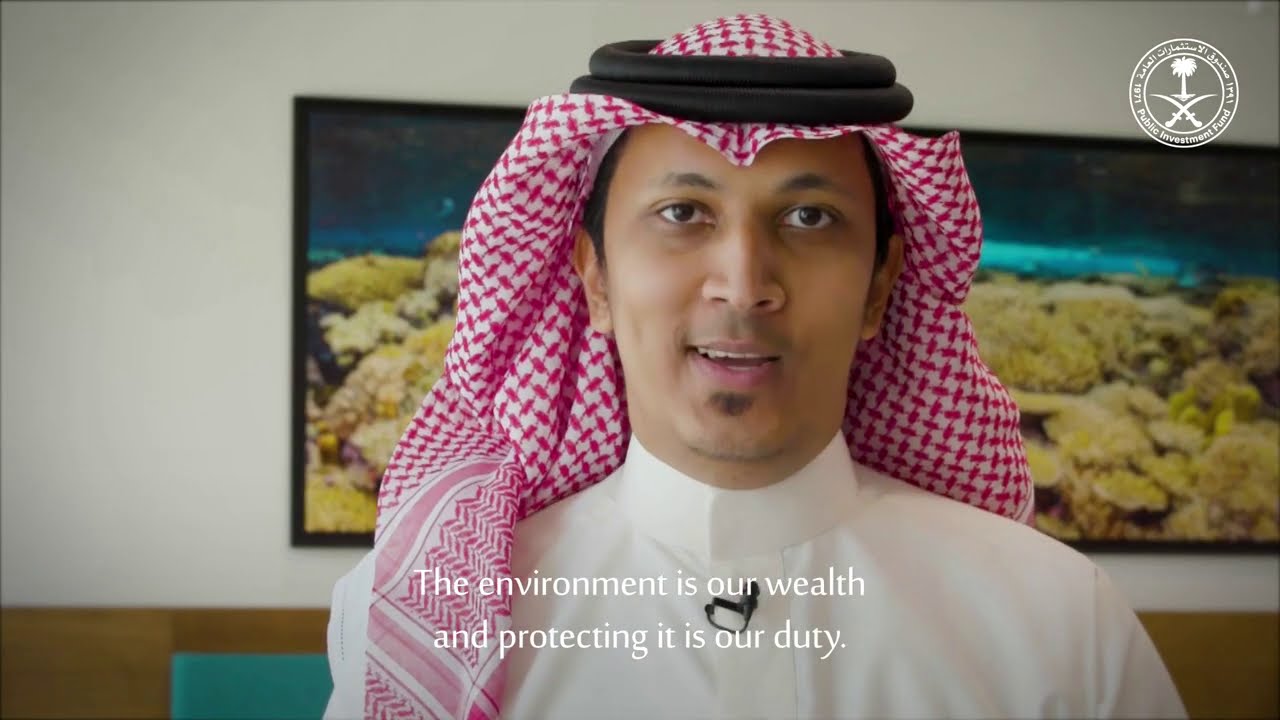The image captures a young man with light brown skin and dark brown eyes, facing the camera and speaking. He wears a red and white Saudi-style headdress with two black circular bands (likely an agal) securing it in place. His short black eyebrows and a small soul patch under his lower lip are visible as he speaks. He is dressed in a high-collared white shirt, with a microphone clipped to it. The camera angle is at chest level, pointed slightly upwards. Behind him, a built-in wall display shows an image of a vibrant coral reef, resembling either an aquarium or a flat-screen TV projection. The upper right corner features a government seal or circular logo, while text at the bottom of the scene reads, "The environment is our wealth and protecting it is our duty."